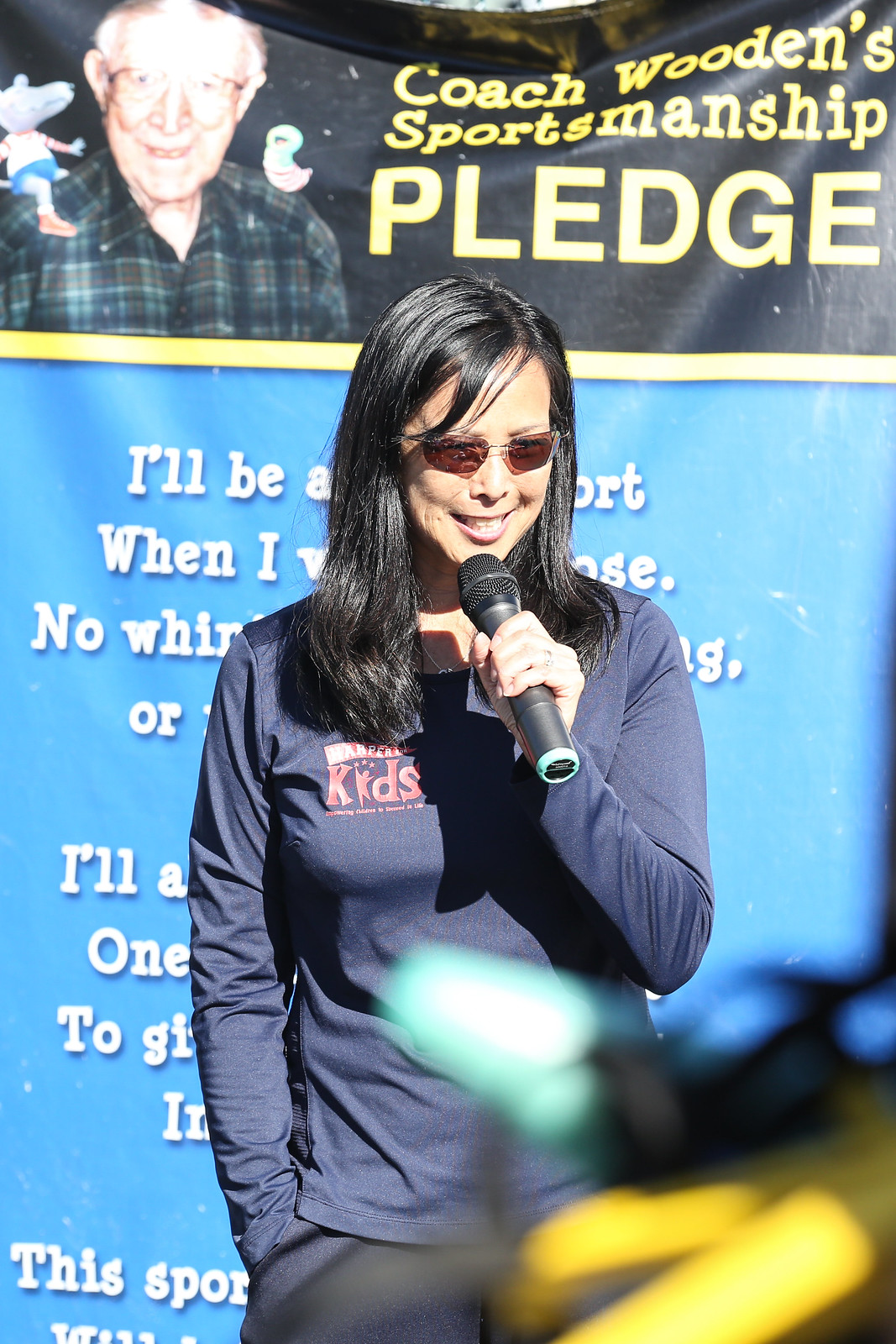In this photograph, a young woman stands under the bright sun, holding a microphone close to her mouth as she speaks to an outdoor audience. She has shoulder-length black hair, tan skin, and is wearing sunglasses, a long-sleeved navy blue spandex shirt, and black pants. Behind her is a prominent powder blue vinyl banner with white lettering, part of which reads "Coach Wooden's Sportsmanship Pledge." The banner also features a photograph of an older man wearing glasses and a plaid flannel shirt. The text on the banner seems to encourage being a good sport and possibly includes a quote or pledge. The event appears to be related to sportsmanship, possibly a fundraiser or kids' sports event, and the woman seems to be an important speaker, engaging the audience with her message.